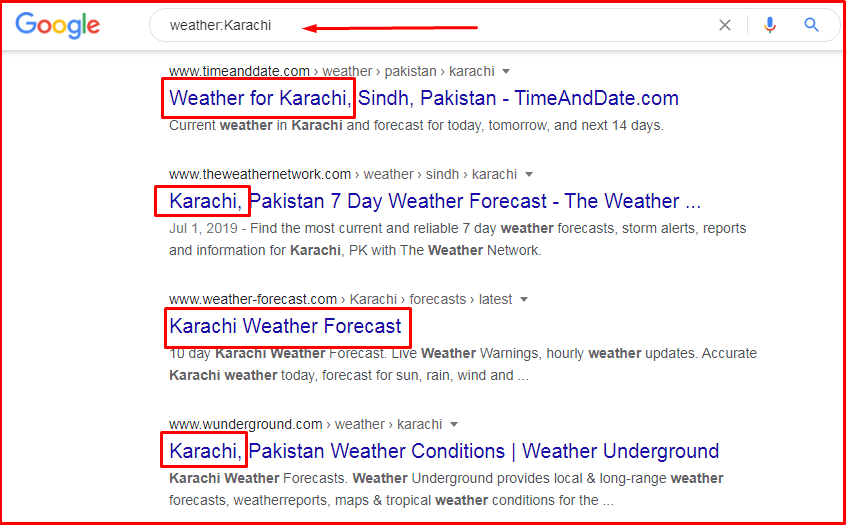A screenshot taken from Google search reveals a white background bordered by a red square. In the upper left-hand corner, the Google logo is displayed in its signature color sequence: blue, red, yellow, blue, green, and red. Within the white search bar, the query "weather, Karachi" is typed in black text, highlighted by a red arrow pointing at it. To the left of the search bar are icons for an 'X' to delete the text, a microphone for voice input, and a magnifying glass for search.

Below the search bar, the first result shows "www.timeanddate.com/weather/Pakistan/Karachi" in black text, enclosed in a red square. The link text itself, "Weather for Karachi", is in blue. The following results include "theweathernetwork.com", "weather-forecast.com", and "Wunderground". Each displays "Karachi" in blue text, highlighted within red squares. These search results provide a range of weather information sources for Karachi.